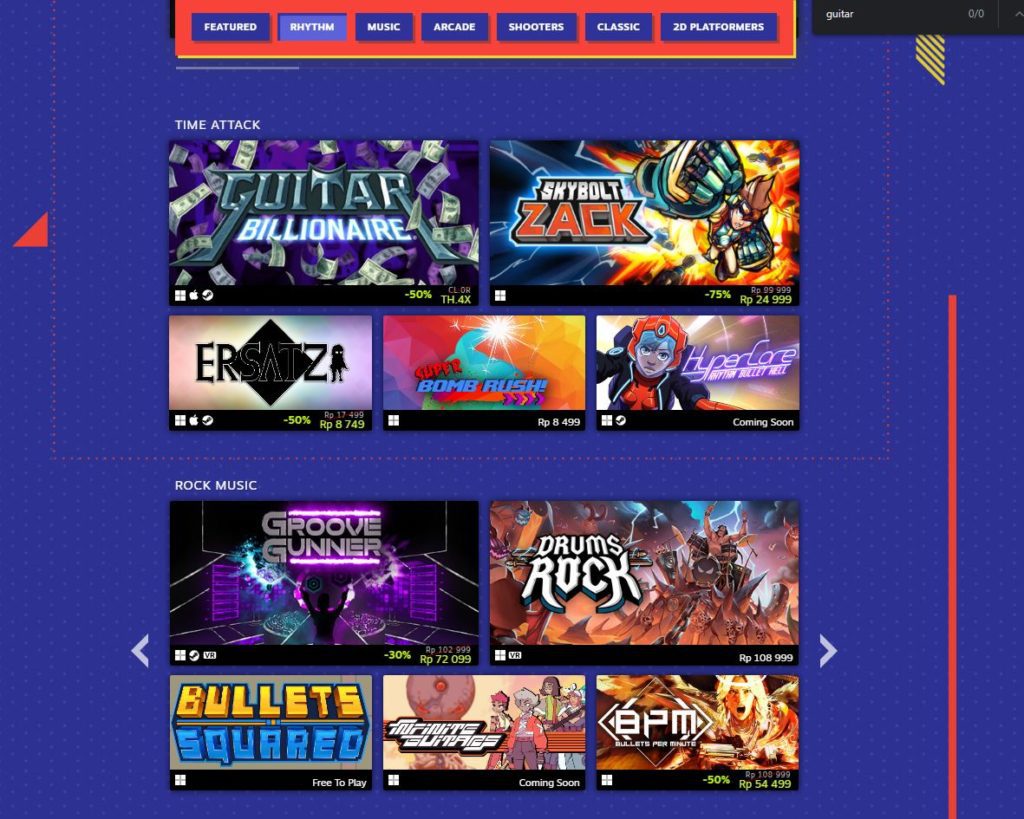**Web Page Screenshot: Gaming Portal**

This screenshot captures the interface of an unidentifiable website with a vibrant and intricately detailed design. 

The background features a bright purple hue enriched with subtle, tiny polka dots of a slightly lighter shade, making for an engaging and textured visual. At the very top center of the page is a prominent red rectangle serving as the navigation menu. The menu itself contains several purple rectangular buttons, each with menu items written in clean white text. From left to right, the menu items include: Featured, Rhythm, Music, Arcade, Shooters, Classic, and 2D Platformers, indicating that this is a gaming-related site.

Just beneath the menu, we find the headline "Time Attack," followed by a layout showcasing five different game images. The top row features three games: "Guitar Billionaire," "Skybolt," and "Zach." Below, three smaller images display additional games: "Airsots," with its title written inside a black diamond in black text, "Bomb Rusk," set against a blue flame-like background, and "Hyper Care."

Further down the page, there's another headline, "Rock Music," introducing a separate game section. This section displays more games: “Groove Runner,” “Drums,” “Rock,” “Bullets Squared,” and another game with an unreadable title. “Bullets” is highlighted in large gold capital letters while “Squared” stands out in large blue capital letters. The final game on the right is titled "BMP," featuring an image of a woman with blonde hair, wearing black lipstick, and with her mouth wide open, adding a dramatic touch to the visual.

The overall design and content suggest this web page is dedicated to showcasing various video games, categorized by genre and themes.